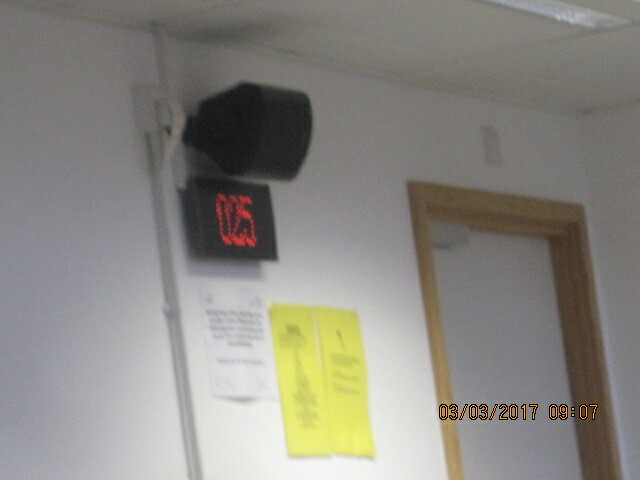This photograph, dated 03/03/2017 at 09:07, depicts a room with a white door framed by light brown wood, likely oak. The door is equipped with a hydraulic piston designed to control its movement. On the left side of the image, a black siren with a white cylindrical attachment is mounted on the white wall. Beneath the siren, glowing red text displays the number "025" alongside a white paper and two rectangular papers with black text, though these are too blurry to read. The ceiling, also white, features rectangular fluorescent lighting. Additional details include visible protective casing for electrical wires running up the wall.